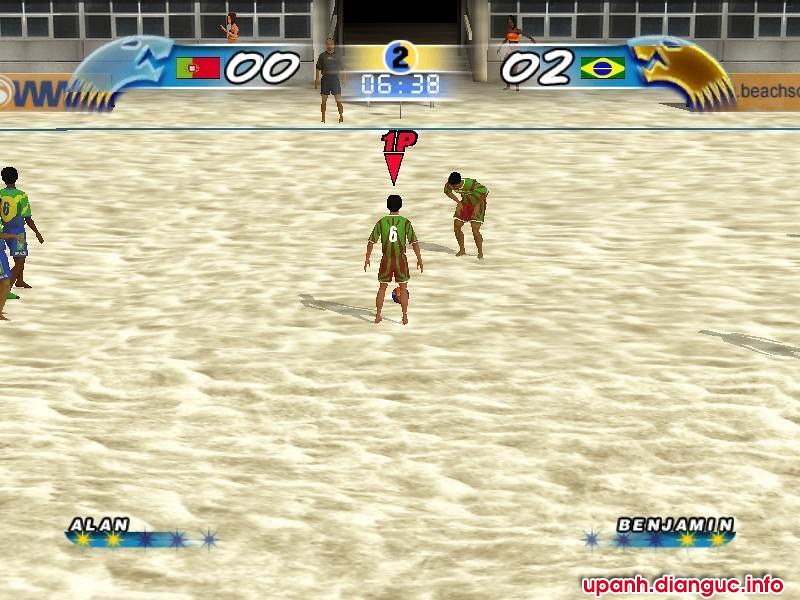This screenshot captures a moment from a video game set in an outdoor, sandy arena. The ground is covered in a sandy texture, indicating a rugged and arid environment. At the center of the scene, there are two players dressed in greenish uniforms with reddish-brown markings. The player in the middle, marked as the first player by a symbol above their head, has a red arrow pointing down at them and is positioned with their back to the camera, suggesting they are in control of their movements. A ball is situated at this player's feet. To the right of the first player, another player donning the same jersey is visible, facing the camera and slightly to the left. This second player is bent over with their hands resting on their thighs, possibly indicating exhaustion or a brief pause in the game.